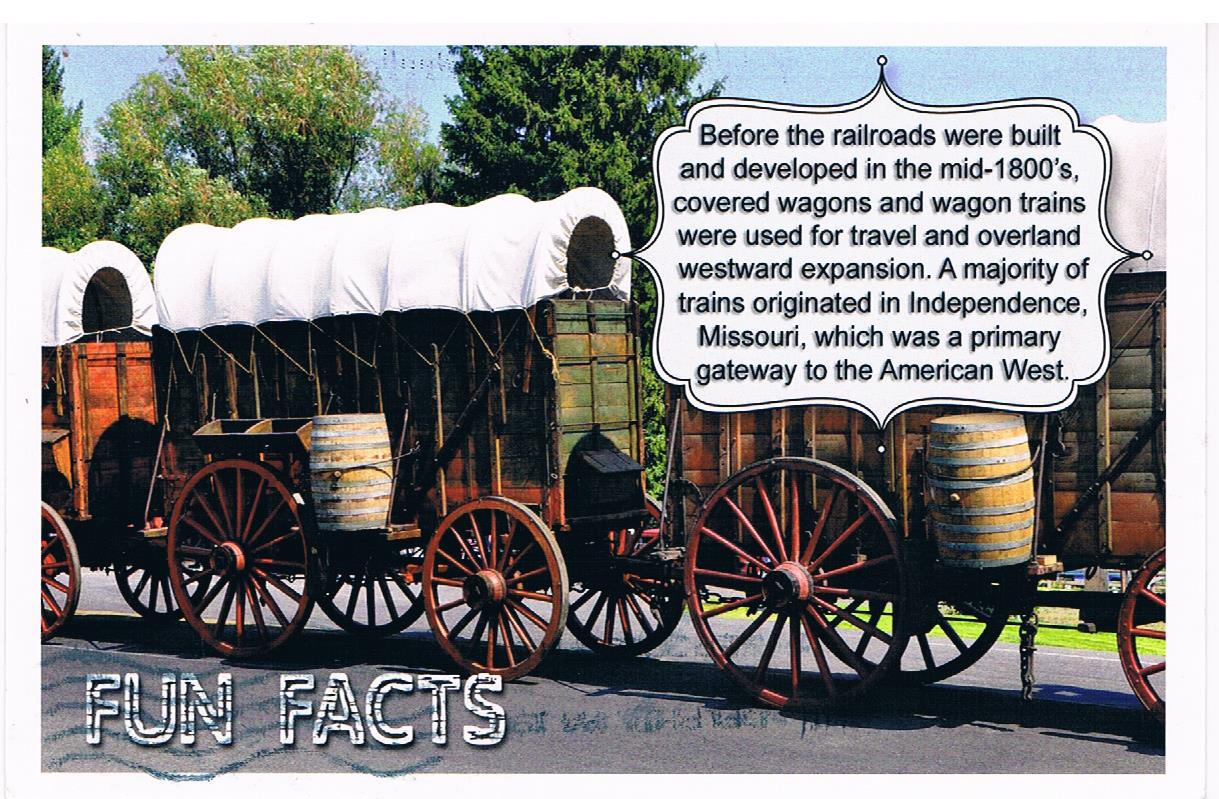This picturesque postcard-like photograph captures a nostalgic scene of historical covered wagons, reminiscent of the era before railroads dominated travel in the United States. The image displays three wooden wagons with striking red-and-black wheels and white canvas coverings, highlighting their robust yet modest design. Each wagon features a brown wooden barrel affixed to its side, suggesting preparedness for a long journey. Set on a concrete ground against a backdrop of a clear blue sky and vibrant green trees—three prominent ones positioned towards the left and center—the scene evokes a sense of outdoor adventure. 

In the upper right-hand corner, a detailed informational bubble proclaims, "Before the railroads were built and developed in the mid-1800s, covered wagons and wagon trains were used for travel and overland westward expansion. A majority of trains originated in Independence, Missouri, which was a primary gateway to the American West." This historical note is framed in a fanciful white-bordered box. The bottom left-hand corner of the postcard features a "Fun Facts" label in white lettering, accompanied by a postmark, hinting at its use for mailing. The image captures the essence of pioneering spirit and the critical role of covered wagons in America's westward expansion.